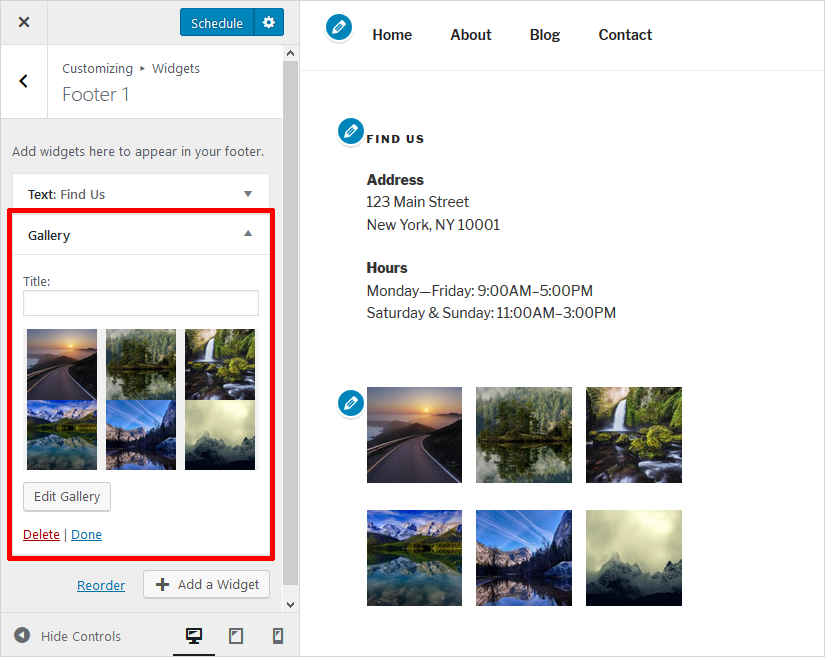The image depicts a web page or app interface with a gray outline, slightly wider than tall by approximately 10-20%. The interface is split into two sections from left to right, with the left section occupying about 35% of the width and the right section taking up the remainder.

**Left Section:**
- The topmost 10% is a gray background. Positioned within this gray area:
  - A black "X" icon is located in the upper left corner.
  - In the upper right, there is a blue "Schedule" button.
  - Additionally, a gear icon for settings is on the far right.
  
- The next 20% contains a white background with the following elements:
  - A left arrow to navigate back.
  - Gray text displaying "Customizing" with a triangle to the right followed by the word "Widgets."
  - Below this, "Footer One" is mentioned.
  
- The rest of the left section has a gray background featuring:
  - The text "Add widgets here to appear in your footer."
  - A "Text" section labeled "Find Us" with a drop-down arrow.
  - A "Gallery" section that includes:
    - An up arrow for a drop-down menu.
    - A title box to be filled in and six placeholder images.
    - An "Edit Gallery" button in the lower-left corner.

The interface is detailed and structured for easy navigation and customization, clearly delineating various sections for widgets and gallery management.